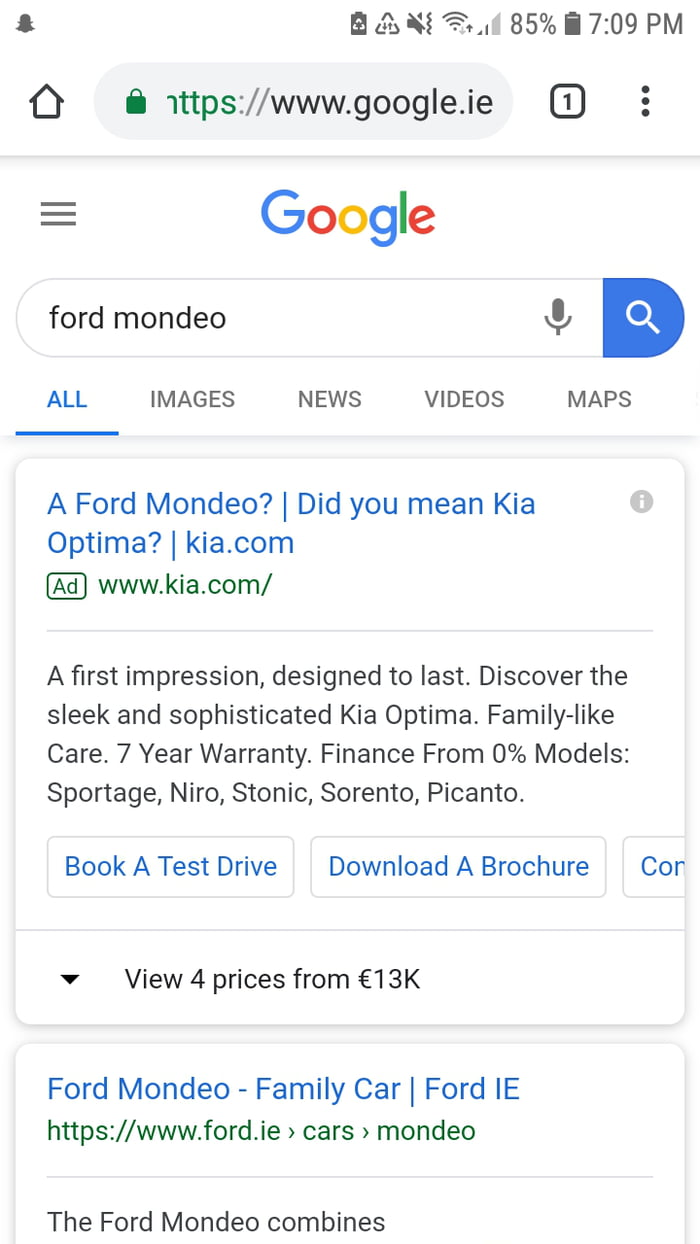A screenshot of a cell phone displays the following details: The time is 7:09 PM, and the battery level is at 85%. The phone has a weak cellular signal with only one bar visible but is connected to a Wi-Fi network with full strength (4 out of 4 bars). The phone is set to silent mode. Two unidentified icons are present in the status bar next to the Wi-Fi and battery indicators. An Instagram notification icon appears in the upper left corner of the screen. Below the status icons is a Google Chrome browser with the URL "google.ie" visible in the address bar, alongside a home button and a vertical three-dot menu icon. Below the address bar, another menu is represented by three vertical lines. The Google logo in its standard colors is prominently displayed, followed by a search bar with the text entry "Ford Mondeo," a microphone icon, and a magnifying glass search button. Search filter options beneath the search bar include "All," "Images," "News," "Videos," and "Apps." A search result asks, "Did you mean Kia Optima?" with a URL link to Kia's official website, Kia.com.